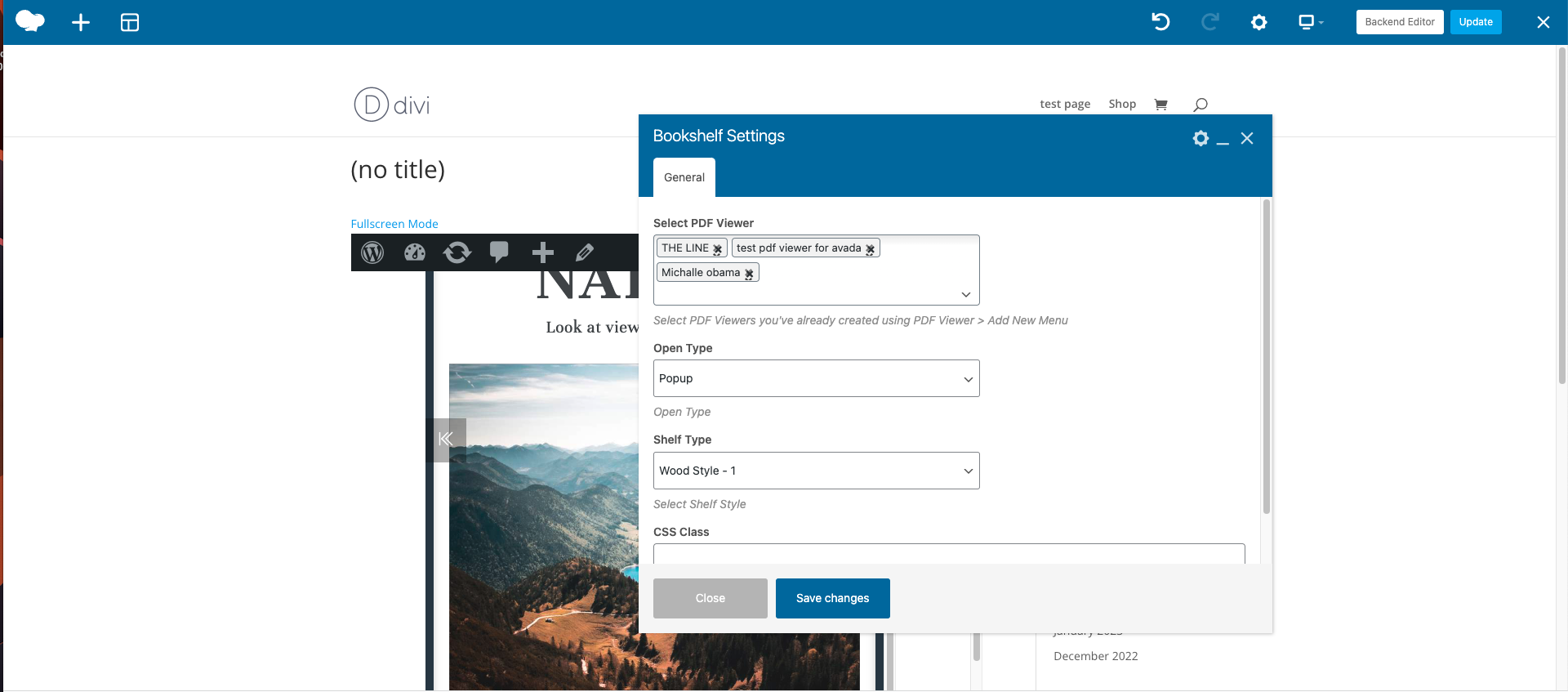In this image, which appears to be a screenshot of a webpage, the header section at the top displays a blue background. Towards the top right corner, there are two buttons: "Backend Editor" in white and "Update" in blue. Additional icons such as refresh, settings, and desktop mode are also visible.

Centrally aligned to the right on the main page, there's a pop-up window titled "Bookshelf Setting," written in white text against a blue background. Below this title, there is a section labeled "General" with a white background. Within this section, the text prompts the user to "Select PDF Viewer," indicating that the selected viewer is "Line Test PDF Viewer for Avada Michael Obama."

Further down, the pop-up provides options to "Select PDF Viewers you have already created using PDF Viewer," and includes an "Add New Menu." The lower part of the pop-up features several settings: "Open Type," which is set to "Pop-up," "Shelf Type," set to "Old Style 1," and an empty field for "CSS Class." At the bottom of the pop-up, there are two buttons: "Close" in grey and "Save Changes" in blue.

In the background of the screenshot, at the top left, the text "DV" is visible, followed by "No Title." Below that, "Full Screen Mode" is indicated in blue text. The rest of the background displays a black WordPress interface. This interface features a distinctive "W" logo at the bottom, along with a graphic of a mountain landscape descending into a blue river, accompanied by dark green trees and brown grass.